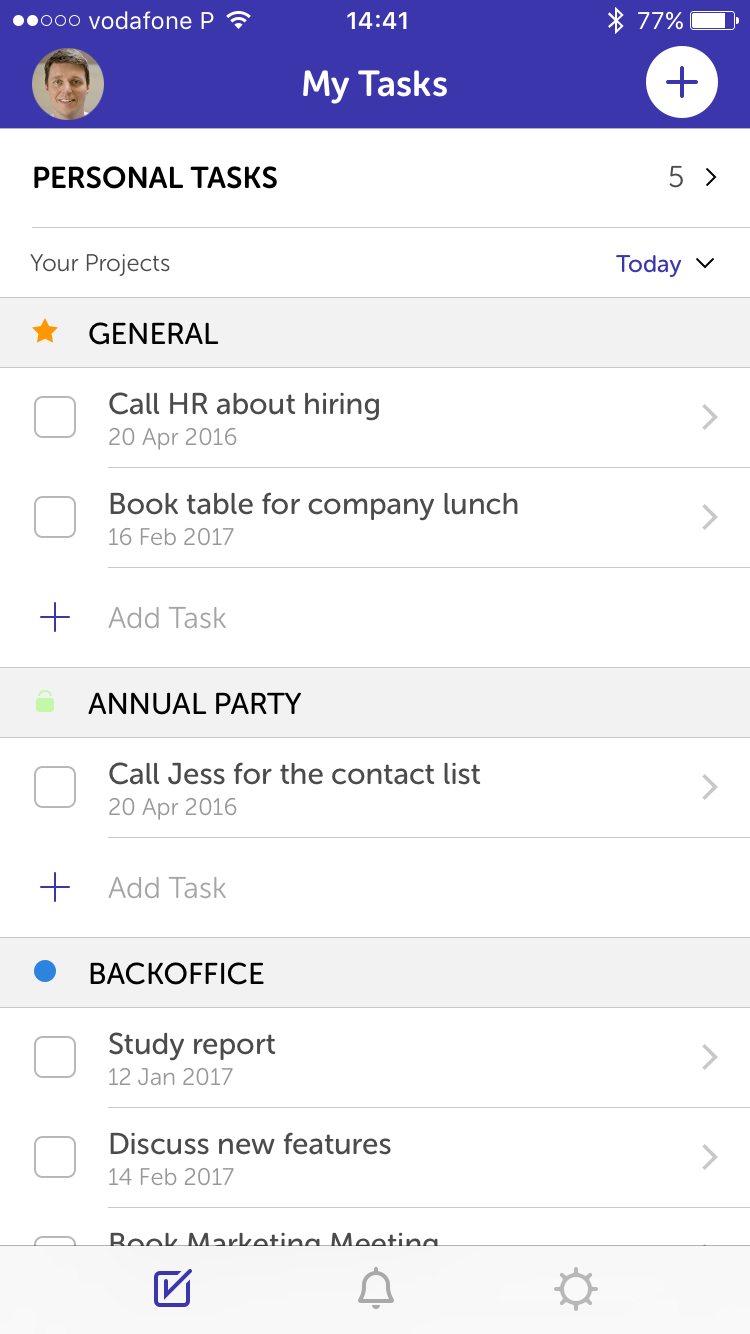A screenshot displays a mobile interface with Vodafone as the carrier. The battery level is at 77%, and the time is 14:41. The task manager is open, showcasing personal tasks, and is titled "My Tasks." 

1. **General (Starred)**
   - Call HR about hiring: Scheduled for April 20, 2016.
   - Book table for company lunch: Scheduled for February 16, 2017.
   - Add task (Plus icon): Annual party (green icon resembling a shopping bag).
   - Call Jess for the contact list: Scheduled for April 20, 2016.

2. **Projects: Back Office (Blue Circle)**
   - Study report: Scheduled for January 12, 2017.
   - Discuss new features: Scheduled for February 14, 2017.
   - Add task (Plus icon): [No task listed].

Additionally, there is a task described as "Book marketing meeting."

The interface highlights ongoing tasks with specified dates, color-coded icons for easy identification, and options to add new tasks.